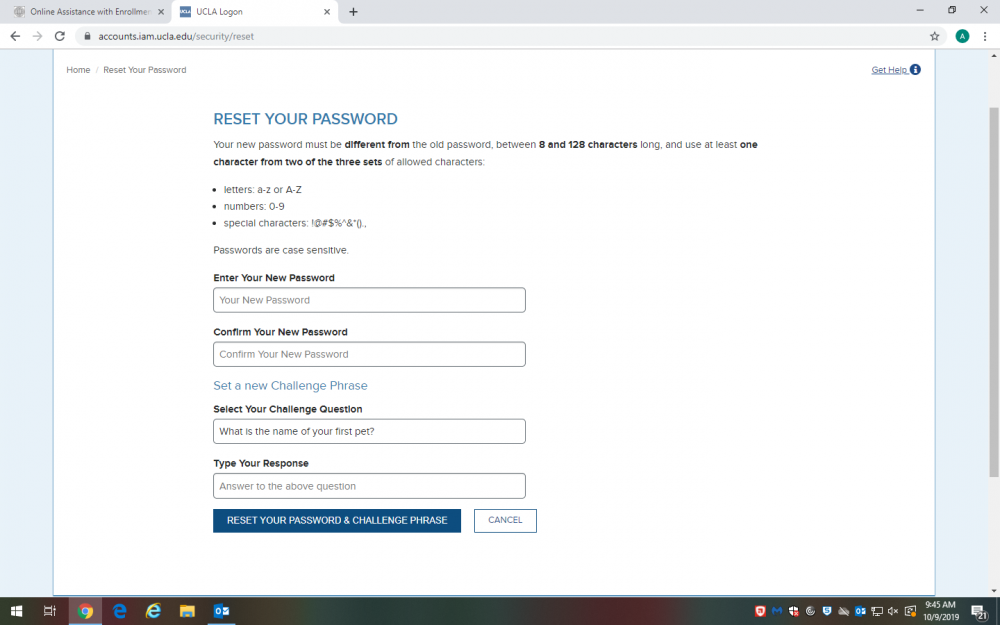A screenshot captures a desktop view with two open browser tabs. The second tab is active, displaying the UCLA Logon page. The URL in the search bar reads "accounts.UCLA.edu," and the page features a clean, white background. 

At the top left corner of the page, options labeled "Home" and "Reset Your Password" are visible. Prominently centered at the top of the page is the heading "Reset Your Password" in bold blue letters, followed by detailed password requirements.

The main content area features two text boxes for the user to input their new password: the first box prompts "Enter your password," while the second requests "Confirm your new password." Below these fields, a section titled "Select a new challenge phrase," in light blue font, introduces additional security steps. Two more text boxes follow, inviting the user to "Select your challenge question" and "Type your response."

At the bottom of the page, a dark blue button labeled "Reset Your Password and Challenge Phrase" appears next to a white button with a blue outline that says "Cancel."